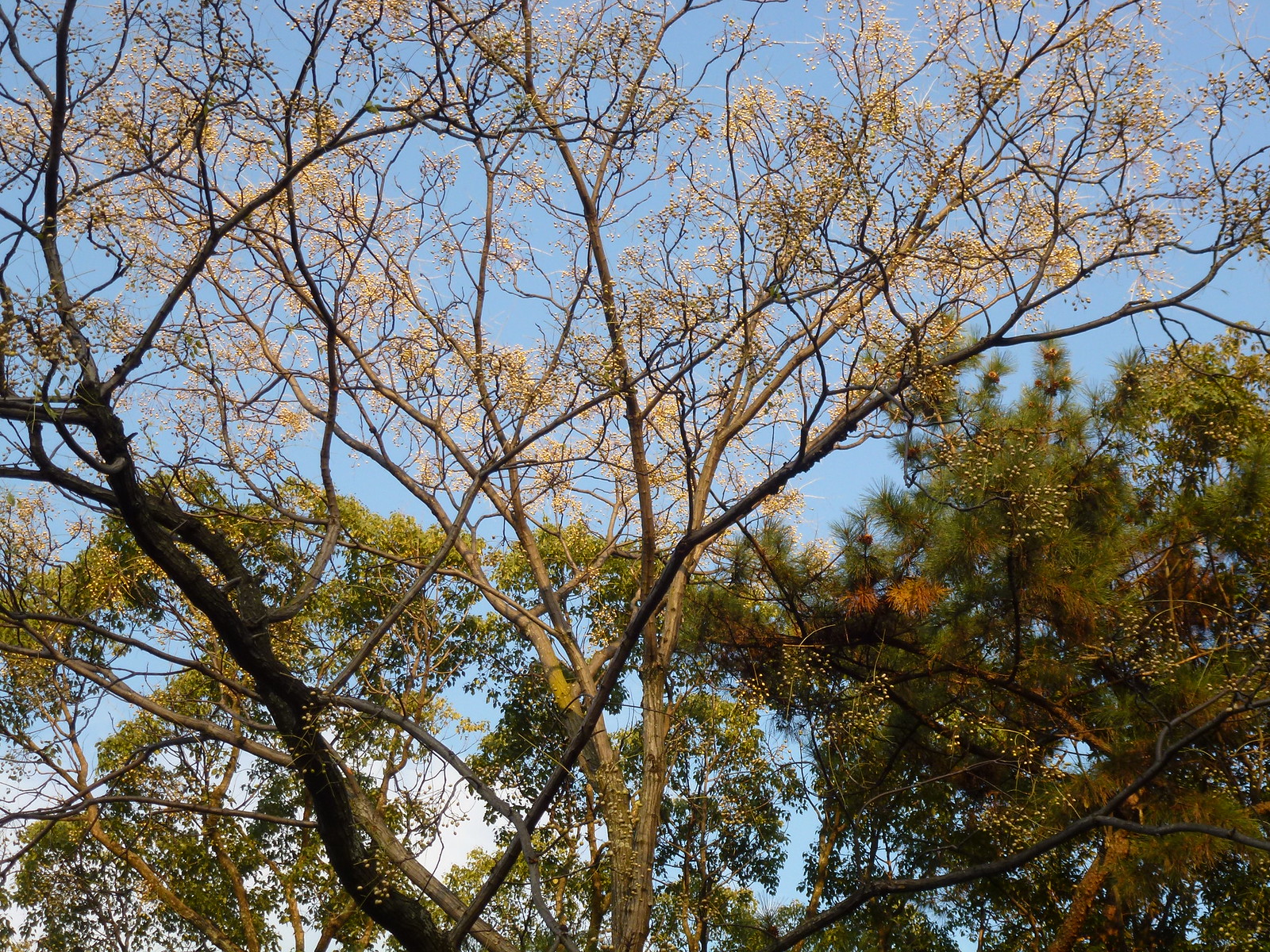The photograph captures a serene daytime scene dominated by the tops of various trees framed against a clear, blue sky. On the left side of the image, a tree with sparse foliage is visible, featuring delicate, yellow flowers that add a touch of color against the azure backdrop. This tree's sparse canopy allows for an unobstructed view of the clear sky behind it. In contrast, on the right side, a noticeably denser tree stands, distinguished by its needle-like leaves. This verdant tree contrasts sharply with its sparser neighbor, providing a rich, green texture to the image. Further adding to the composition, in the lower right corner, another tree (or perhaps multiple trees) with abundant green foliage contributes to the varied tapestry of leaves. The different types of trees and their varying densities of foliage create a layered, detailed landscape that highlights the peaceful beauty of nature.